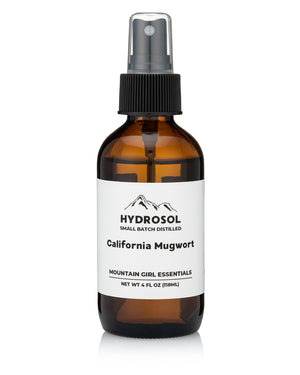This is a product photo showcasing a small, amber-tinted spray bottle with a net weight of 4 fluid ounces. The bottle, made of transparent brown glass, features a black pump spray nozzle protected by a clear cap. There is a black cap beneath the clear protection. The bottle is adorned with a white label that covers three-quarters of its surface. The label is simple, featuring black text that reads "Hydrosol, Small Batch Distilled, California Mugwort, Mountain Girl Essentials." Additionally, the label includes a silhouette of mountains beneath the word "Hydrosol." The photo has a clean white background with a slight reflection or shadow at the bottle's base, enhancing its professional presentation, possibly aimed at product listings on websites or e-commerce platforms.